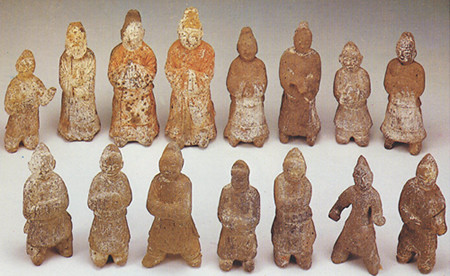The photograph captures a color image of 15 ancient terracotta figurines arranged on a light-colored background. The figures are organized into two distinct rows: the back row contains eight figurines while the front row displays seven. These Chinese-looking figures, varying in height as well as posture, possess a weathered appearance with some adorned in remnants of white paint, while others reveal the original terracotta material. Most of the figurines have their arms folded or clasped in front of them, dressed in robes and topped with various hats. Notably, a few stand out with different arm positions; for instance, one figure in the back row with arms outstretched as if holding a spear or staff, and another in the front row on the far right with outstretched arms. The color palette of these figurines ranges from light brown to dark reddish brown. The photograph, which lacks any additional elements such as people, animals, or structures, draws attention to the fine, albeit worn, details of these historical artifacts.